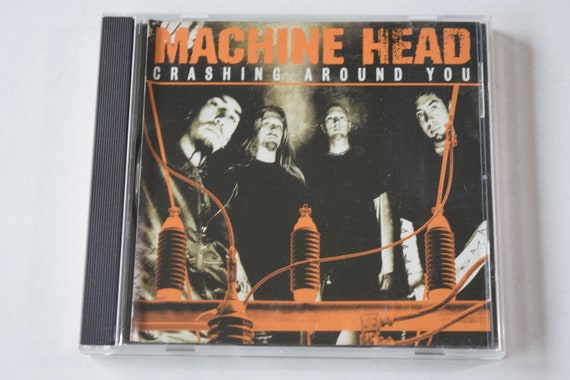This is a photograph of a CD case on a plain white background, featuring a typical 90s-style clear plastic front with a black plastic hinge. The CD is by the band Machine Head, with the album titled "Crashing Around You." The cover showcases the text "MACHINE HEAD" in bold orange letters at the top, with the album title "CRASHING AROUND YOU" in white text beneath it. Below the text line, a black and white photo of the four band members is displayed from left to right. The first member on the left has a black goatee, the second has long blond hair with black streaks and a brown goatee, the third sports very short brown hair and a small blond goatee, and the fourth member on the right has short black hair with a black goatee. At the bottom of the CD cover, there is an image of electrical equipment resembling power line components, featuring three metal cylinders with coils around them. Wires extend from the coils on both sides and one in the foreground with a wire extending up to the left. The electrical components are depicted in an orange variation, providing a striking contrast to the monochromatic photo of the band.